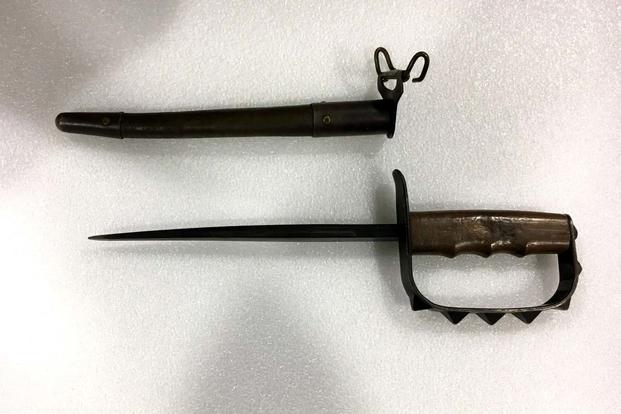The photograph, set against a white, textured background with visible shadows, showcases an antique bayonet with a thick, wickedly sharp black blade. The bayonet features a wooden handle on the right side, intricately adorned with metal dog collar-type studs along the knuckle side, suggesting dual functionality for both slashing and punching. Above the bayonet rests its sheath, likely made of leather, detailed with a metal hook closure that secures it to the blade. The sheath, dark and sturdy with visible screws and a circular metal attachment, complements the weapon. The overall composition provides a detailed look at these historically significant objects, highlighting their craftsmanship and intended use.